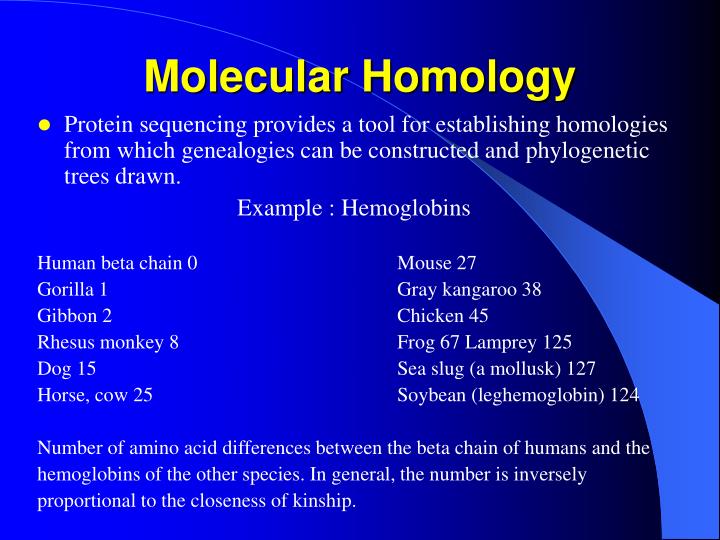The image resembles a slide from a PowerPoint presentation, featuring a blue background. At the top, in yellow font, it reads "Molecular Homology." Below that, in white font, the slide states: "Protein sequencing provides a tool for establishing homologies from which genealogies can be constructed and phylogenetic trees drawn." Following this, an example regarding hemoglobins is given. To one side, it lists: "Human beta chain 0, Gorilla 1, Gibbon 2, Rhesus Monkey 8, Dog 15, Horse 25, Cow 25." Opposite, it continues: "Mouse 27, Gray Kangaroo 38, Chicken 45, Frog 67, Lamprey 125, Sea Slug (a mollusk) 127, Soybean (leghemoglobin) 124." At the bottom, it further clarifies: "Number of amino acid differences between the beta chain of humans and the hemoglobins of other species. In general, the number is inversely proportional to the closeness of kinship."